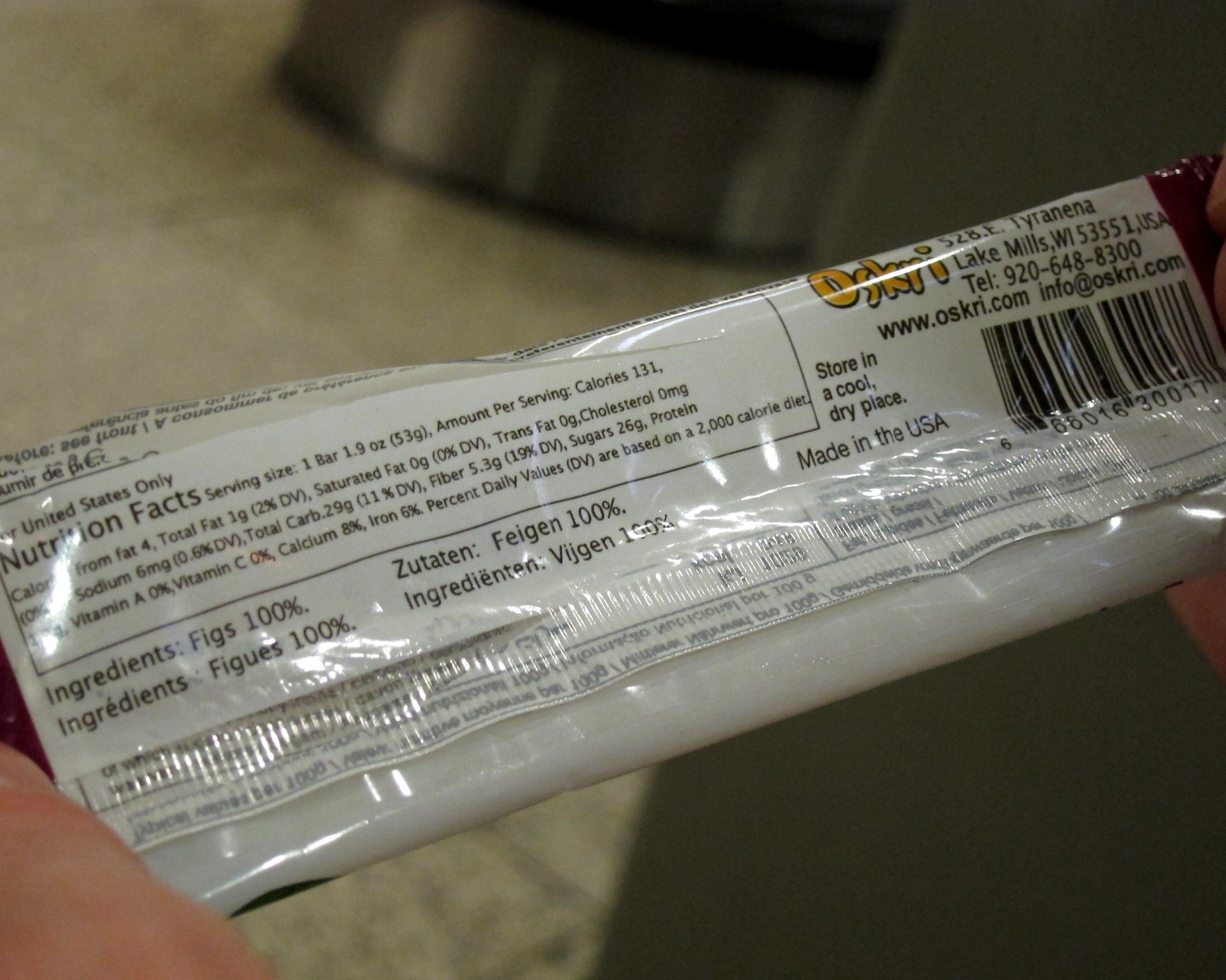This image captures the back of an Oskri fig bar wrapper, prominently held up by a finger in the bottom left corner, with a portion of another hand slightly visible on the right. The wrapper is primarily white with black text outlining the nutritional facts and ingredients under a reflective layer of plastic. Key details include the brand name "Oskri" in yellow text at the top, their website www.oskri.com, and the ingredient list specifying "figs 100%". Information about the product specifies it is made in Lake Mills, Wisconsin, USA with a detailed barcode on the right side of the wrapper. The wrapper also states "Store in a cool, dry place" and mentions the contact number 920-648-3300. The image background shows a section of a floor with white, tan, and black tiles, and a bit of a tan wall, indicating a domestic indoor setting.